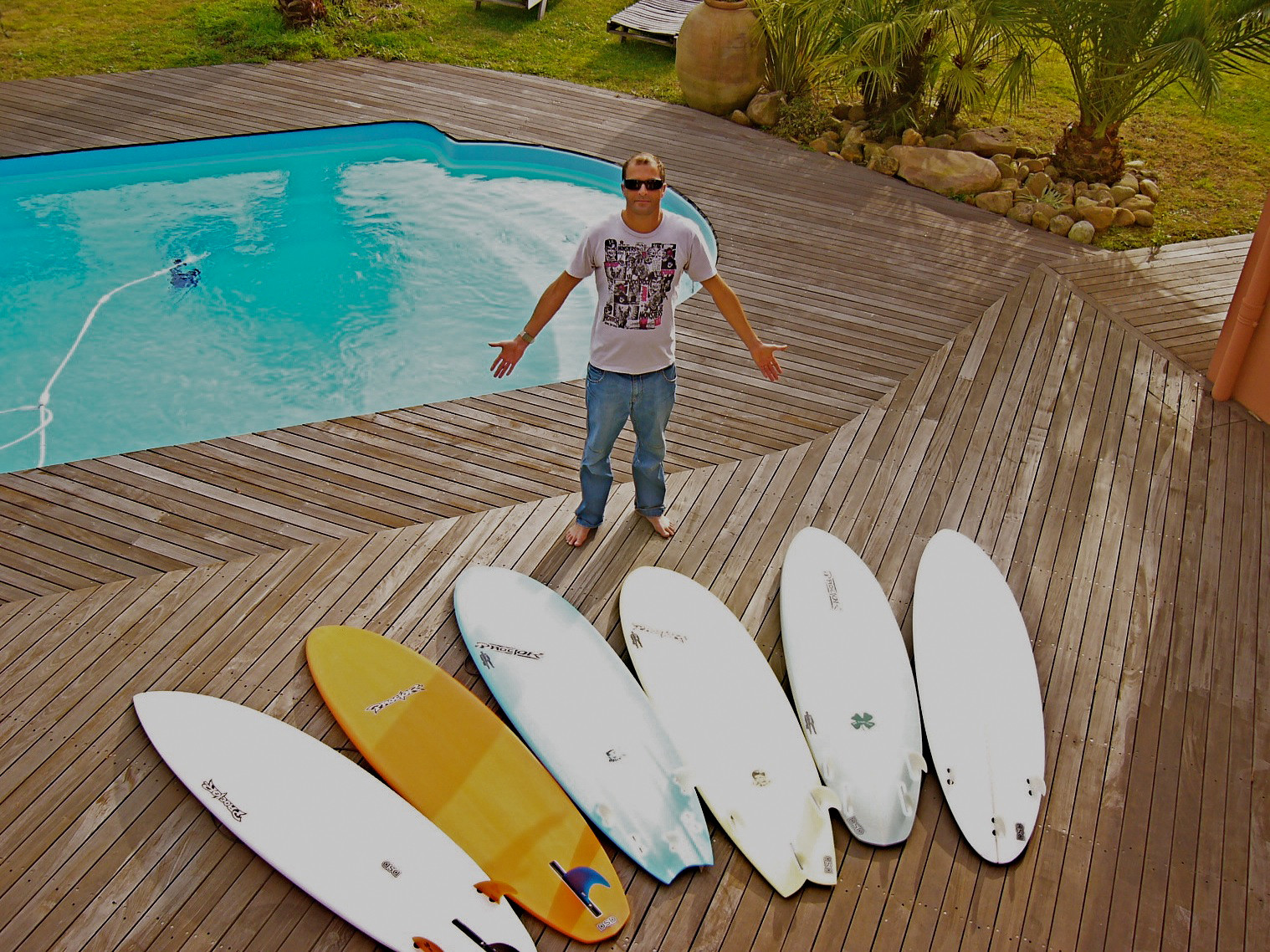The image features a fair-skinned man standing poolside on a paneled wooden deck. He is barefoot, dressed in blue jeans and a white t-shirt adorned with a graphic design that resembles a QR code. The man’s arms are outstretched, revealing a watch on his left hand, and he is wearing sunglasses. Arranged neatly in front of him on the deck are six surfboards, all facing up with visible fins. Five of the surfboards are predominantly white, while the second one from the left is adorned with blue and orange hues. The first surfboard has red fins, and the second has a blue fin.

The pool behind him is clean and bright blue, featuring steps for easy entry. Visible in the pool are some white tubing and a blue device. Beyond the pool, the scene extends to a few planted trees surrounded by decorative rocks, a patch of grass, and some lawn chairs. Additionally, short palm trees are visible towards the upper right corner of the image, enhancing the luxurious ambiance of the area. No one else is present in the scene, emphasizing the man's contemplative stance as he surveys the surfboards.